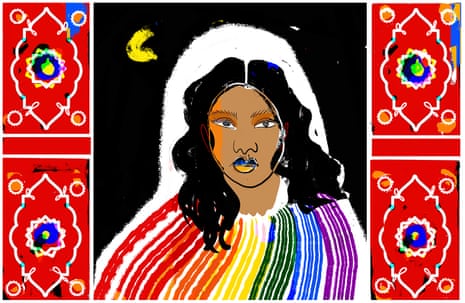This image is a captivating square painting that features intricate, symmetrical patterns and a striking central figure. Each side of the painting is bordered by two red squares, each containing a design that resembles a leaf flanked by small round circles. Inside the leaf-like outline are hues of yellow, blue, and green, slightly resembling a shield or emblem. These red squares are stacked vertically, adding a balanced repetition to the composition.

The center of the painting is a dramatic black background, highlighting a black woman with a serene expression. She has long black hair, parted in the center, and a soft white halo subtly accentuates her form. Her attire is a vibrant multicolored shirt adorned with horizontal stripes in shades of red, white, orange, yellow, green, blue, and purple. Adding to the night-like background, a yellow crescent moon graces the upper left corner, blending elements of nature and human beauty in this artistic tableau.